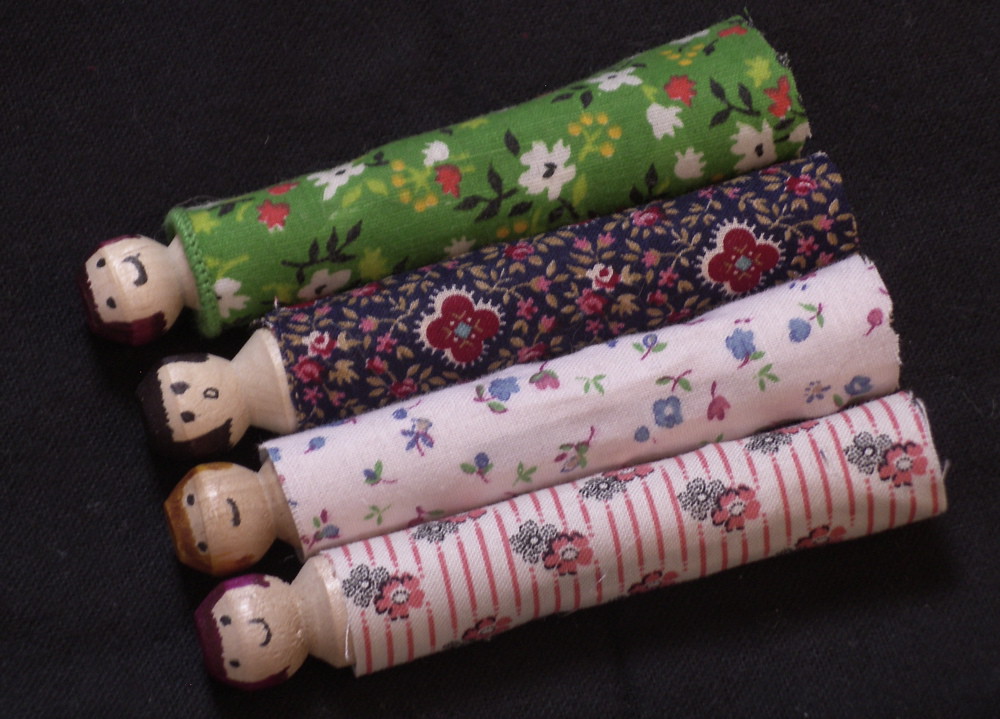This photograph displays four cylindrical wooden dolls, each adorned with unique facial features and wrapped in vibrant fabrics. The dolls, lying atop a tightly knit black mat, have meticulously painted faces characterized by two black dots for eyes and smiles. The hair color of the dolls varies: the ones on the ends have purple and dark purple hair, while the two in the middle sport auburn and light brown hues. Starting from the left, each doll is wrapped in a distinctive piece of fabric. The furthest left wears a vibrant green fabric decorated with white flowers; next is a doll in deep blue cloth adorned with red and pink floral patterns. The third doll is cloaked in pink fabric with contrasting blue flowers, and the fourth wears a white cloth with pink and gray flowers, embossed with pink stripes. Each doll's unique attire and detailed facial expressions add a charming personality to this meticulously arranged display.